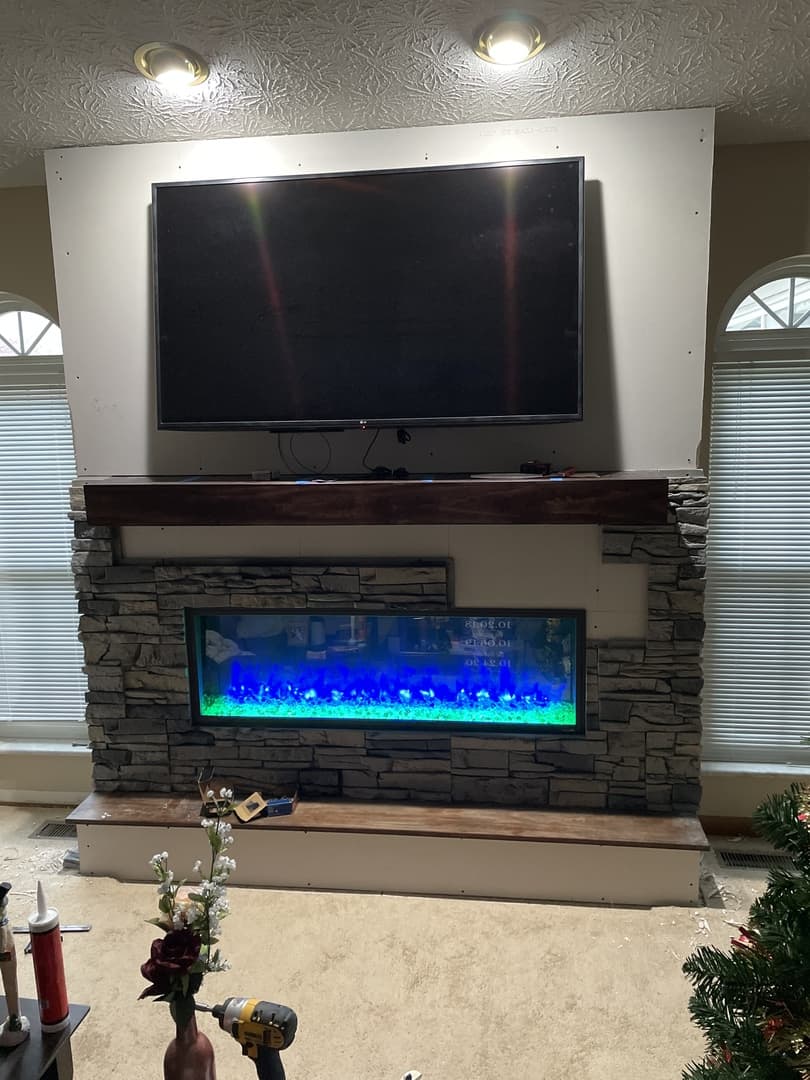The image depicts a detailed view of a cozy living room. Dominating the scene, a large flat screen TV is mounted on a white wall above a faux fireplace with a sophisticated stone veneer finish. The fireplace is framed by a rich, dark brown polished wood mantel, adding a touch of elegance. Inside the fireplace, a digital display showcases vibrant, neon-like flames in shades of blue and green behind a glass screen with a sleek black frame, lending a modern touch.

Flanking the fireplace are two arched windows adorned with white blinds, letting in subdued light. Below the TV, the stone facade of the fireplace features brown bricks, although some parts reveal white drywall behind the veneer, indicating ongoing renovations. The short, light brown carpet adds warmth to the space.

To the right of the fireplace, a Christmas tree adds a festive charm, while on the left, a black table holds a variety of items including a tool that appears to be a yellow and black screwdriver, and a vase filled with red, white, and purple flowers. The ceiling, adorned with patterns and recessed lighting, is white with a popcorn texture. Altogether, the room exudes a blend of modernity and homeliness, capturing an inviting, slightly work-in-progress living space.